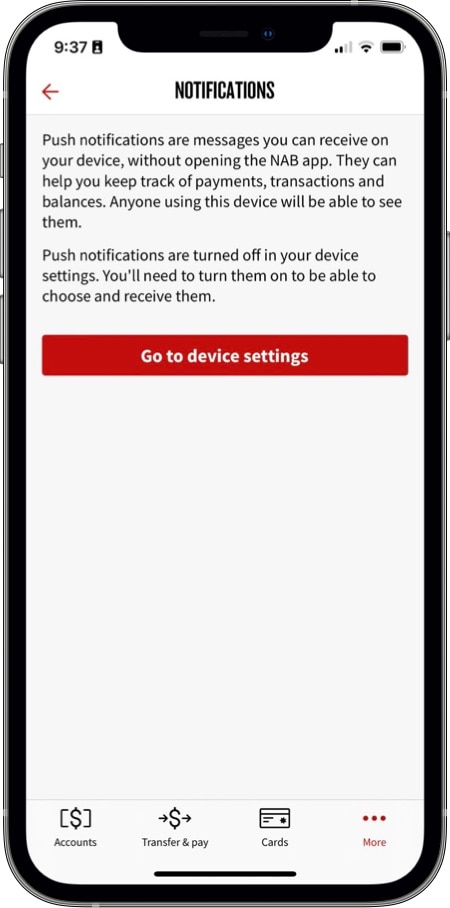Here is the cleaned-up, detailed caption:

"A detailed screenshot of a smartphone interface featuring a notification settings screen. The smartphone is encased in a sleek black bezel. At the upper right corner, the display shows the current time as 9:37 in a black font. Adjacent to the time, there is a small square icon. Along the top right corner, status icons indicate the device's connectivity: the mobile signal shows 2 out of 4 bars, the WiFi signal displays 2 out of 3 bars, and the battery icon is shown as fully charged.

Beneath these indicators, on a white screen, bold black text states 'Notifications,' accompanied by a red arrow pointing to the left.

Further down, on a slightly grey-toned white background, black text reads: 'Push notifications are messages you can receive on your device without opening the NAB app. They can help you keep track of payments, transactions, and balances. Anyone using this device will be able to see them. Push notifications are turned off in your device settings. You’ll need to turn them on to be able to choose and receive them.'

Below this informational text, a red rectangle button with white font instructs 'Go to Device Settings.' The lower portion of the screen is largely empty, creating a clean and uncluttered look.

At the very bottom, there is a row of four icons: a square with a dollar sign on the far left, a dollar sign encircled by arrows to its right, followed by a credit card icon, and finally, three vertical black dots on the far right."